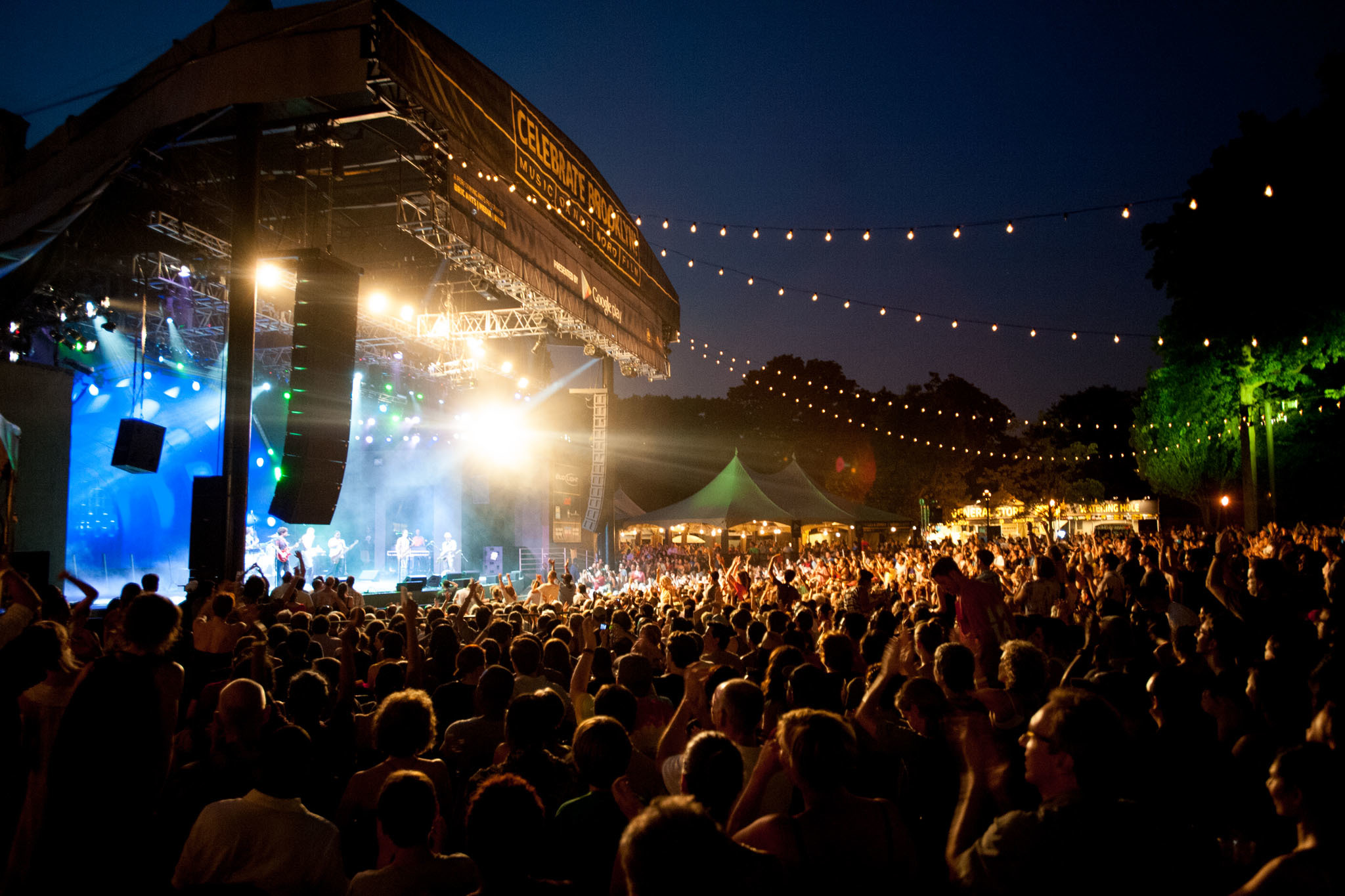The image depicts a vibrant nighttime concert scene. The sky is extremely dark, highlighted by the silhouette of distant mountains and a large, bright green tree positioned on the back right side. The stage, situated to the left of the image, is large and juts out to the right, covered with a big black awning and decorated with strings of lights extending from its top, disappearing into the distance. The stage features a prominent banner with partially legible gold writing that begins with "Celebrate."

Illuminated by an array of bright lights, the stage radiates a vibrant blue hue, casting light onto the performers, including guitarists and keyboardists, who number at least six or seven. The performers are small and lack fine detail due to the photo being taken from the perspective of someone far back in the audience. A large screen behind them displays a similarly bright blue color. Below, a massive crowd, likely numbering in the hundreds, extends from the middle of the image all the way off the frame to the right. Many in the crowd have their hands raised in enthusiasm. 

To the right of the stage, in the background, tents are visible, also illuminated by lights, along with a conspicuously lit building. Some parts of the crowd remain in darkness due to their distance from the stage lighting. The entire scene is a bustling, dynamic depiction of an open-air concert, capturing the energy and atmosphere of the night.